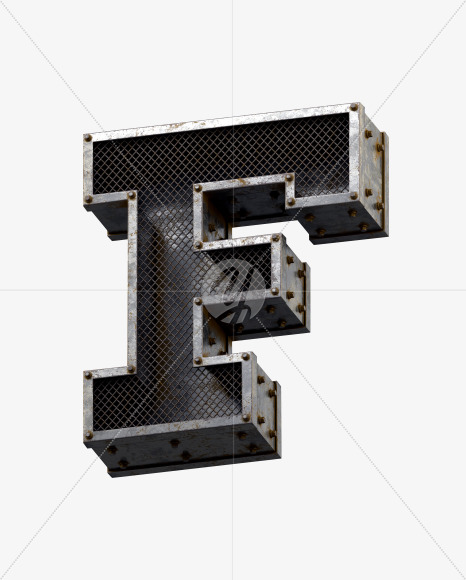The image is a black and white photograph depicting a large, three-dimensional, capital letter "F" made of metal. The background is light gray with faint lines and a watermark with the letter "Y" in the middle. The "F" is outlined in metal, showing signs of rust and age, particularly on the sides where the rust appears brown. The front of the letter features a white mesh overlay, resembling a cage or fence, allowing a view of the dark interior. Each corner of the "F" has a metallic bolt, and additional bolts on the sides, each surface having bolts arranged symmetrically—four on the three sides facing right and six on the bottom. The metallic edges and bolts give the "F" a sturdy, industrial appearance.